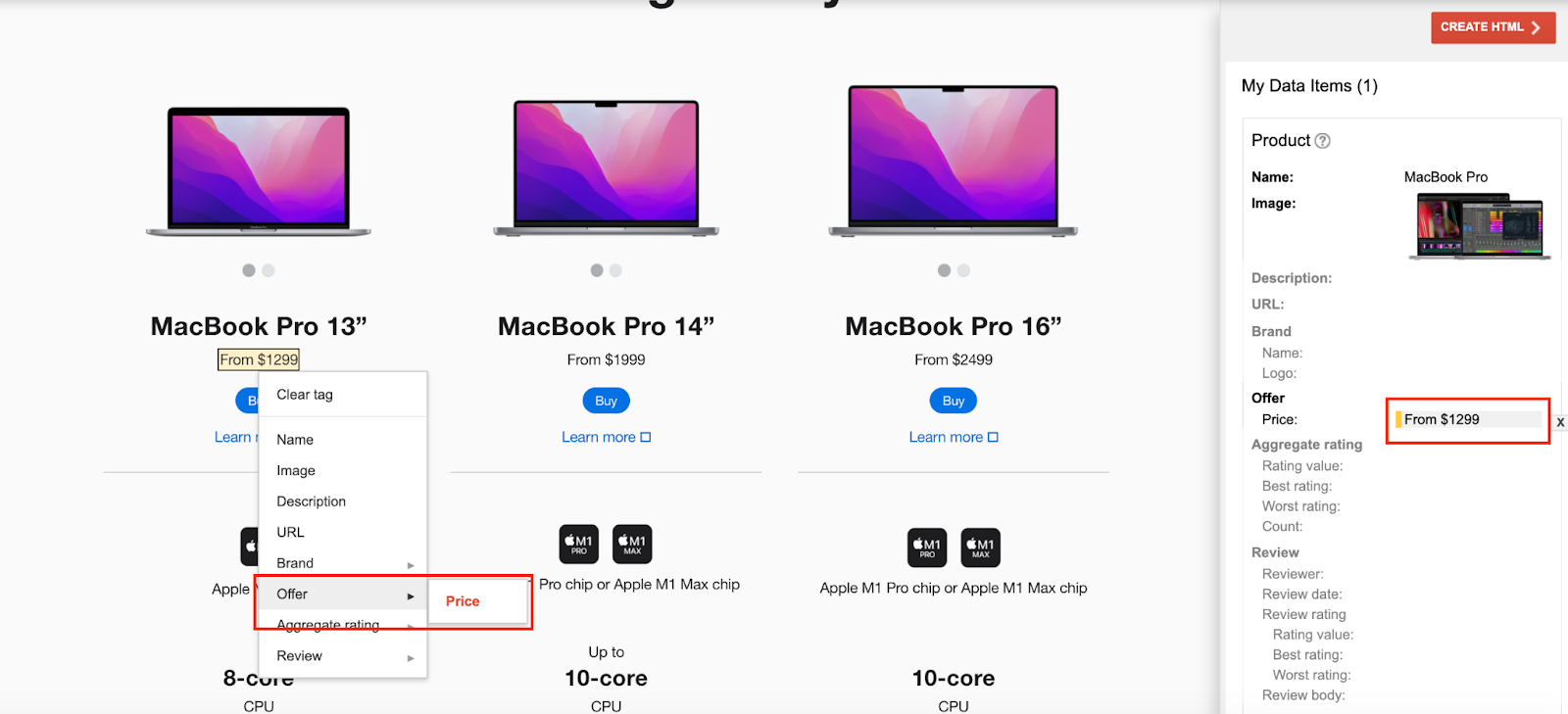The image showcases a webpage displaying details about the MacBook Pro in three different screen sizes: 13 inches, 14 inches, and 16 inches. On the right side of the page, there is a column labeled "My Data Items," featuring sections for product name, image, description, offer, aggregate rating, and review. The offer for the MacBook Pro is prominently highlighted, starting from $1,299 for the 13-inch model. The pricing for the other models is also displayed: $1,999 for the 14-inch MacBook Pro and $2,499 for the 16-inch version. The 14-inch model offers options for either the Apple M1 Pro Chip or the Apple M1 Max Chip, while the 16-inch model includes either the Apple M1 Pro Chip or the Apple M1 Max Chip. The price for the 13-inch MacBook Pro is highlighted in red, emphasizing its starting point of $1,299.